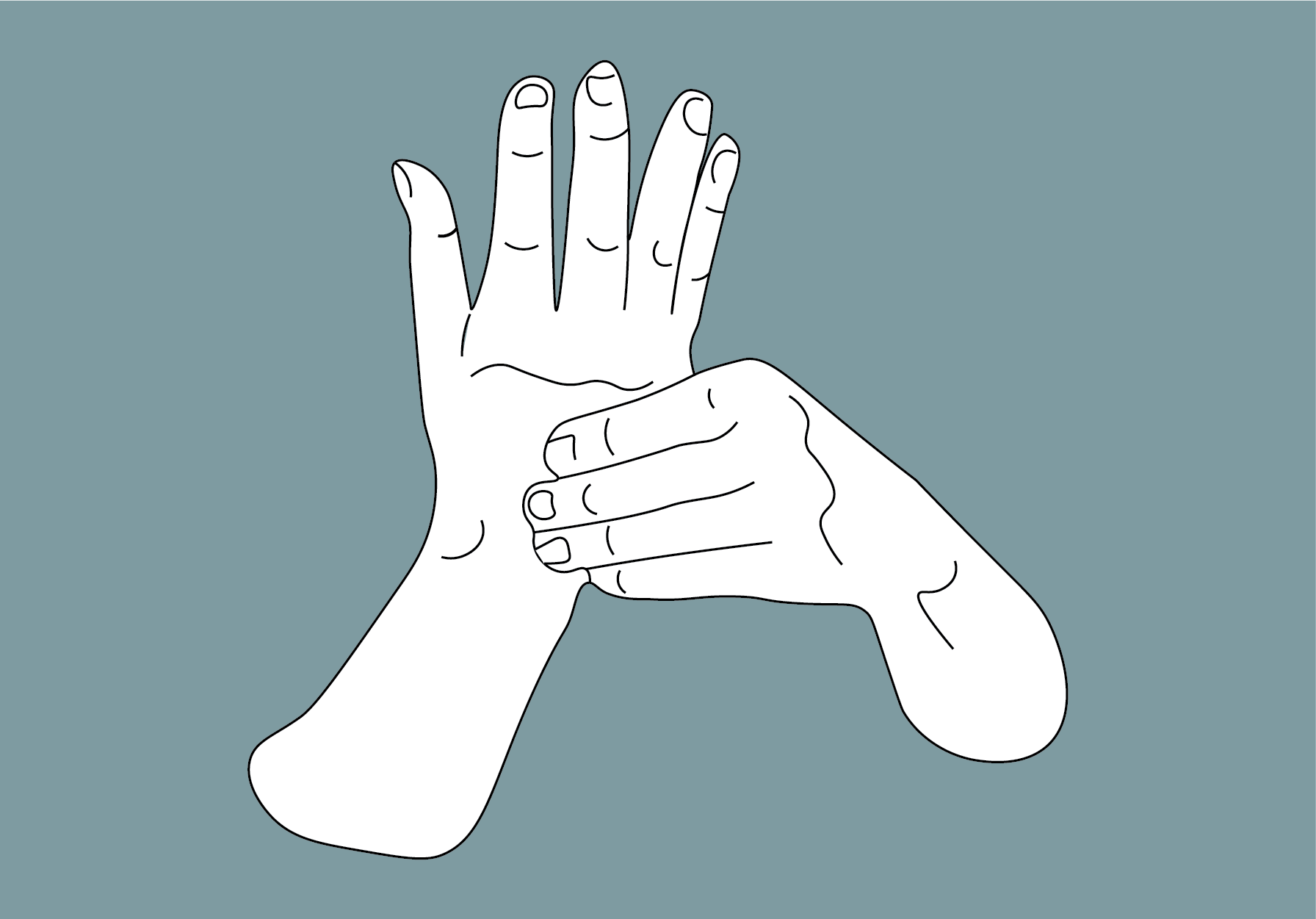The image showcases a detailed black and white line art illustration of two hands set against a dark aqua background. On the left side of the image, the back of the right hand is prominently displayed, extending from the fingers down to the lower part of the arm, displaying several small lines on the fingers and a longer wavy line below. The right hand is in a vertical position, with fingers pointing upwards and spread apart. On the right side of the image, the left hand is depicted as massaging the right hand, with its four fingers pressing on the back of the right hand near the top. The left thumb is not visible. Intricate details like the fingernails on each finger and subtle lines enhance the realism of the illustration. The wrist of the right hand extends downward to the bottom left area, completing the depiction of a massage technique.